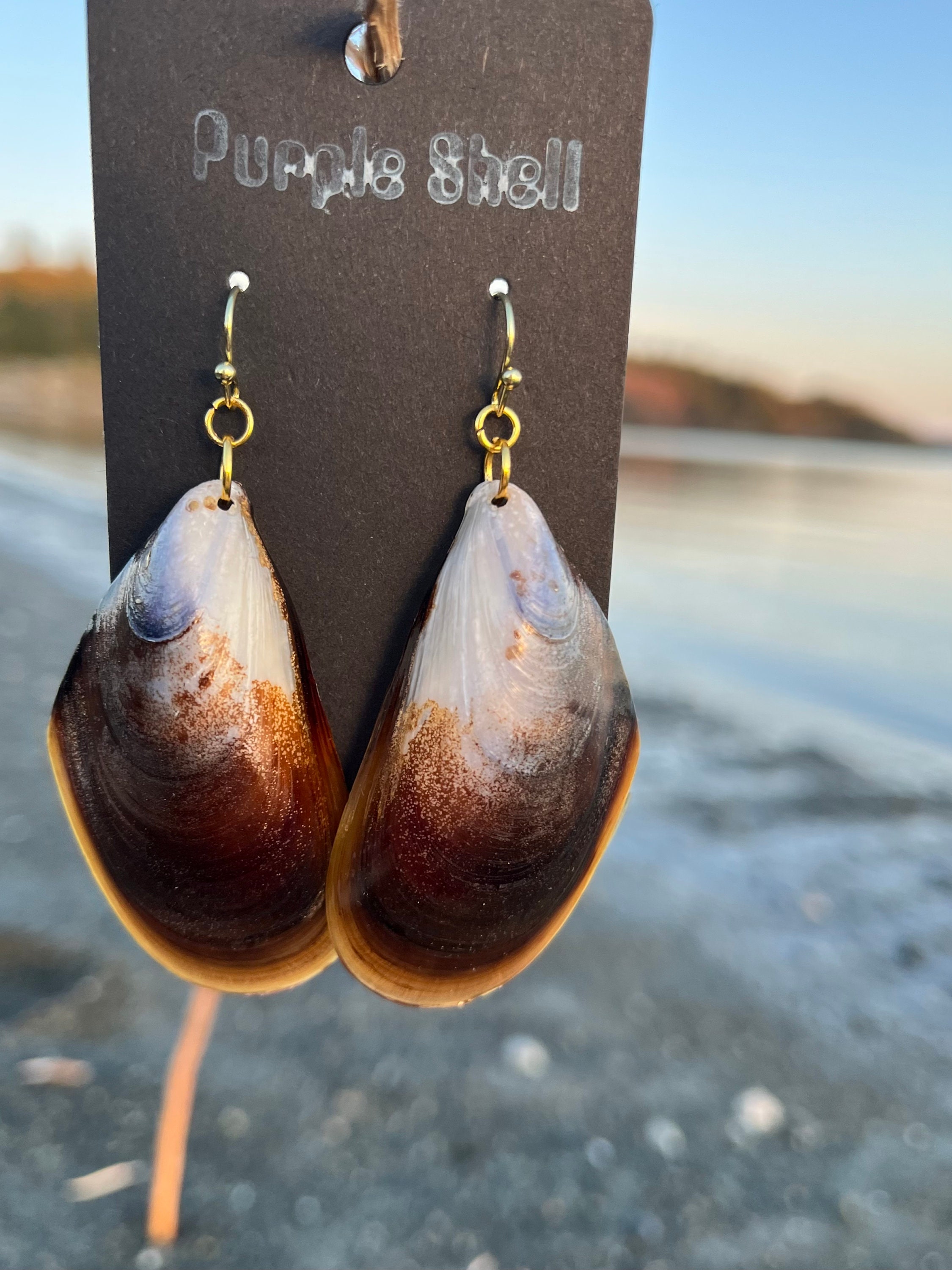In the foreground of this image, a pair of intricately designed shell earrings hang from a piece of brown cardboard labeled "Purple Shell" in white lettering. The earrings feature real shells, each with a light blue and white upper section transitioning to a darker brown at the bottom, and are equipped with small gold loops for wearing. The cardboard appears to be mounted on a stick that is embedded in the ground. The background, slightly blurred to keep the focus on the earrings, is set against a serene beach scene. A calm expanse of water is framed by a peninsula with a gentle hill rising from it. The sky, suggesting either a late afternoon or evening, arches above the scene. The ground is strewn with darker earth mixed with rocks, shells, and other debris, giving the beach a rugged, natural look rather than the typical sandy appearance.